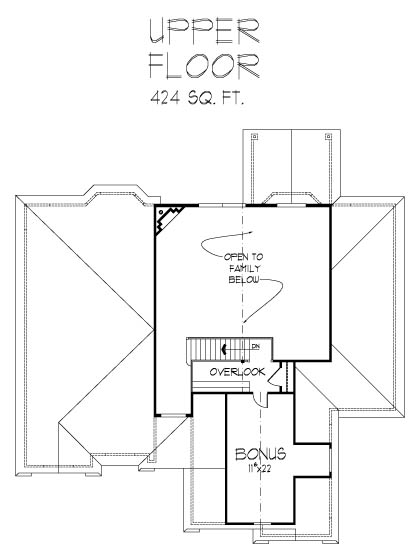This architectural drawing depicts the upper floor of a home, meticulously rendered in black and gray on a white background. At the top center, the drawing is labeled "Upper Floor" across two lines, with the text "424 SQFT." situated directly below this title.

The primary image illustrates a top-down view of the home's layout, which is predominantly square in shape. Various lines traverse the drawing, delineating distinct sections and rooms. 

At the precise center of the image, there is a square room with a small extension, remarkably reminiscent of the letter "P". This area is annotated with "Open to Family Below," framed by squiggly lines above and below the text. Directly beneath this space, a set of stairs is indicated, with an arrow directing to the left.

Adjacent to these stairs is a rectangular area marked "Overlook," which features door symbols. Further below is another rectangular area, labeled "Bonus, 11' x 22'." This space includes a dotted line running vertically from the top to the bottom end of the bonus room, presumably indicating an optional or flexible wall placement.

On the left and right sides of the drawing, two additional rectangular spaces are outlined. The detailed design shows a light gray outline encircling all these shapes, representing the walls of the upper floor.